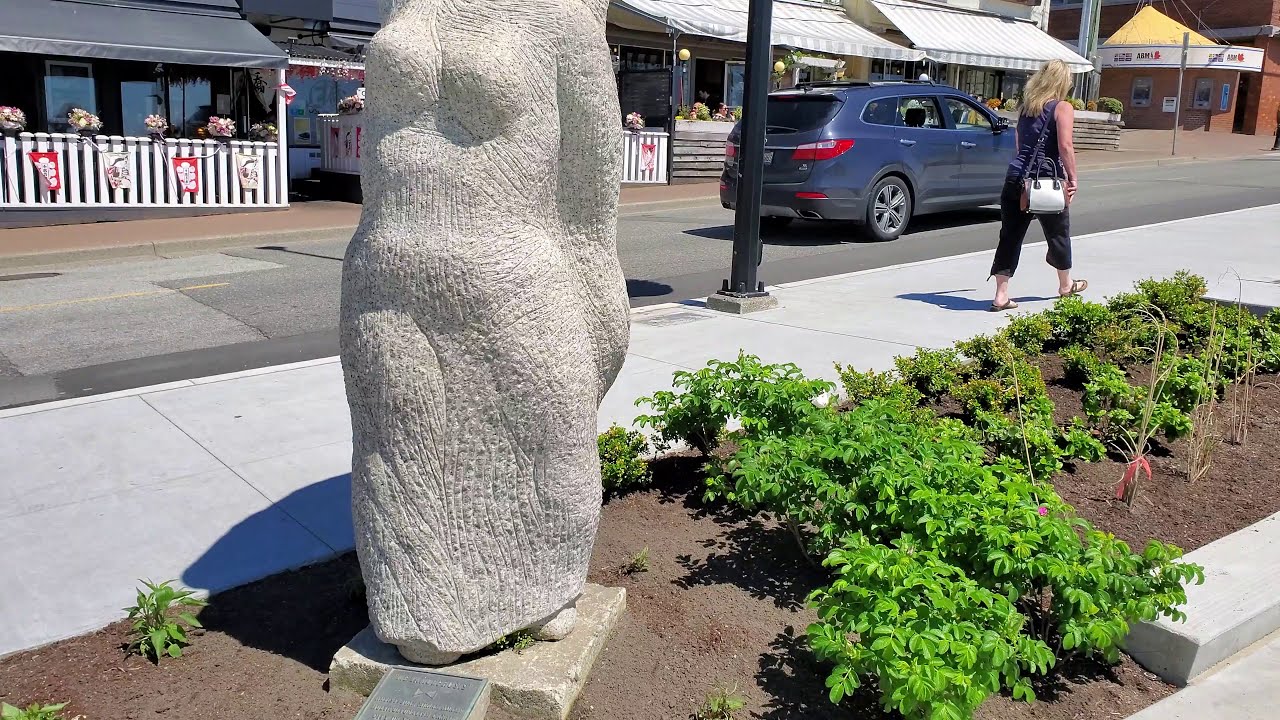In this bright, sunny photograph taken in what appears to be a small city, the scene features a bustling street lined with various shops and restaurants adorned with awnings, patios, and flower arrangements. The main focal point in the foreground is a sizable stone sculpture with a vaguely humanoid, possibly female form, standing about six to seven feet tall in a small patch of dirt beside the sidewalk, surrounded by short green plants. On the sidewalk to the right, a woman with blonde hair, dressed in a blue outfit and sandals, and carrying a white purse, walks past the sculpture. The road next to the sidewalk is paved and features a blue four-door station wagon driving by. A sunny day casts shadows to the left, adding to the lively, inviting atmosphere of the street.